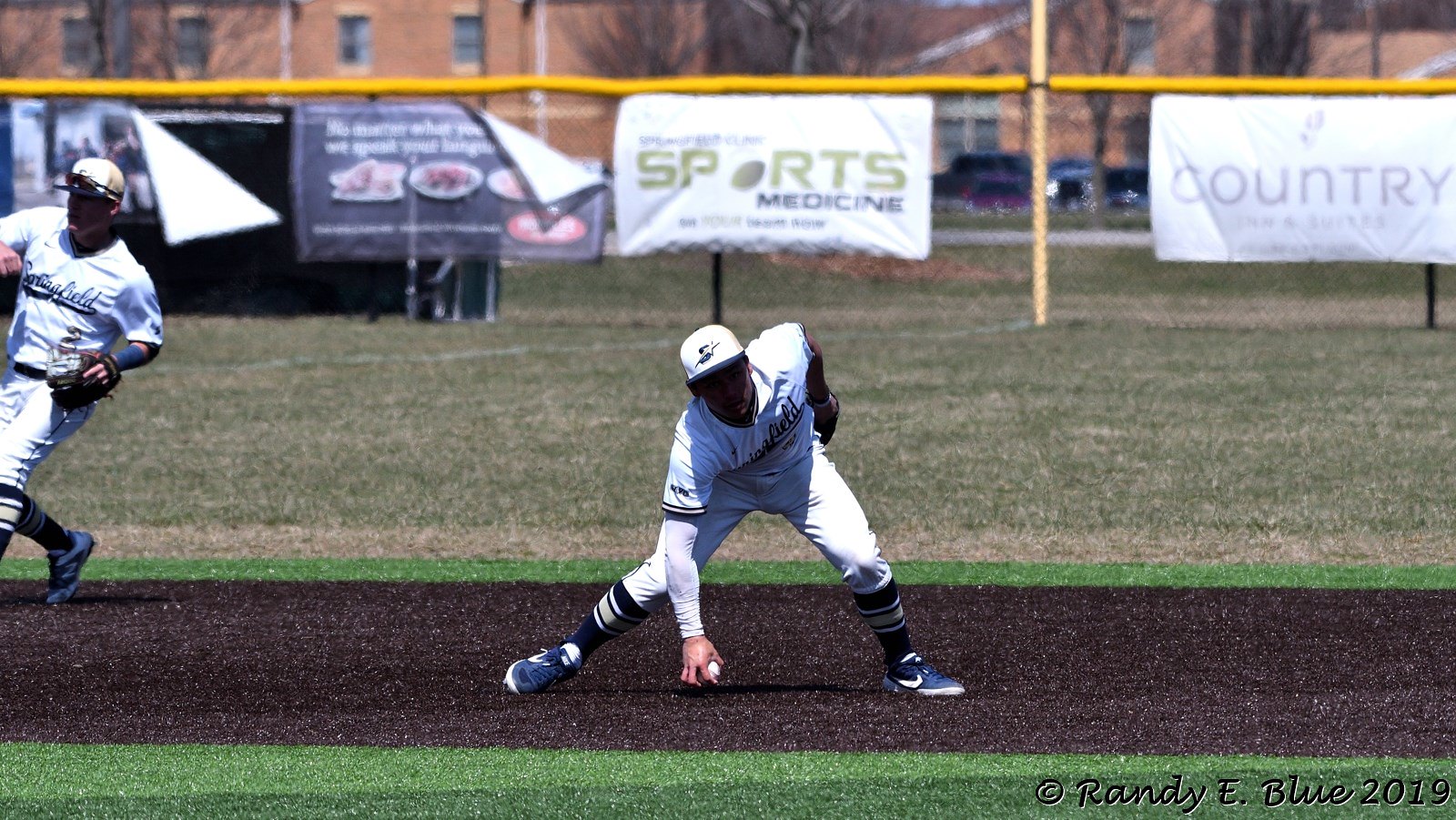The photograph captures a bright, sunny day during a baseball game. Two players from the same team, dressed in white uniforms with white caps, are positioned in the outfield area of the green baseball field. The player in the center is kneeling down to pick up a baseball, with his other hand positioned on his back. Meanwhile, another player is seen running nearby, dressed in an identical uniform. Both wear additional black socks and blue sneakers. The background features an iron fence with a yellow strip of padding on top, intended for safety in case players need to jump and balance while making a catch. The fence is adorned with various sponsorship banners, some of which are partially detached and in need of re-hanging. Behind the fence, a parking area and a series of blurry red brick buildings are visible. The primary colors in the scene are the green of the grass and the white of the uniforms, with some black and blue details adding contrast. The bottom right corner of the image is marked with "copyright Randy E. Blue 2019".